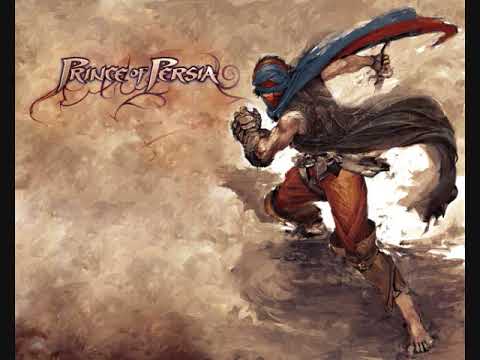The image appears to be a blurry screenshot of a website on a computer screen, likely related to the video game Prince of Persia. The background is predominantly solid black with accents of blue, creating a dark ambiance for the page. At the top, the text "Prince of Persia" is prominently displayed, with a banner underneath that reads, "Discover the Xbox 360 achievement chosen by fans." The text is primarily in white, some of which has a blue outline.

On the top left corner, the Ubisoft logo is faintly visible, while the top right corner contains menu settings that are too distorted to discern. In the middle of the image, the URL "princeofpersia.uk.ubi.com" is written in white font. Additionally, there's an incomplete text below this URL stating, "I'll post it in the description box that way I think," followed by a series of dots and an arrow, suggesting this might be a screen grab from a video tutorial or walkthrough. Throughout the image, there are various small, blurry images and distorted text, making specific details difficult to decipher.